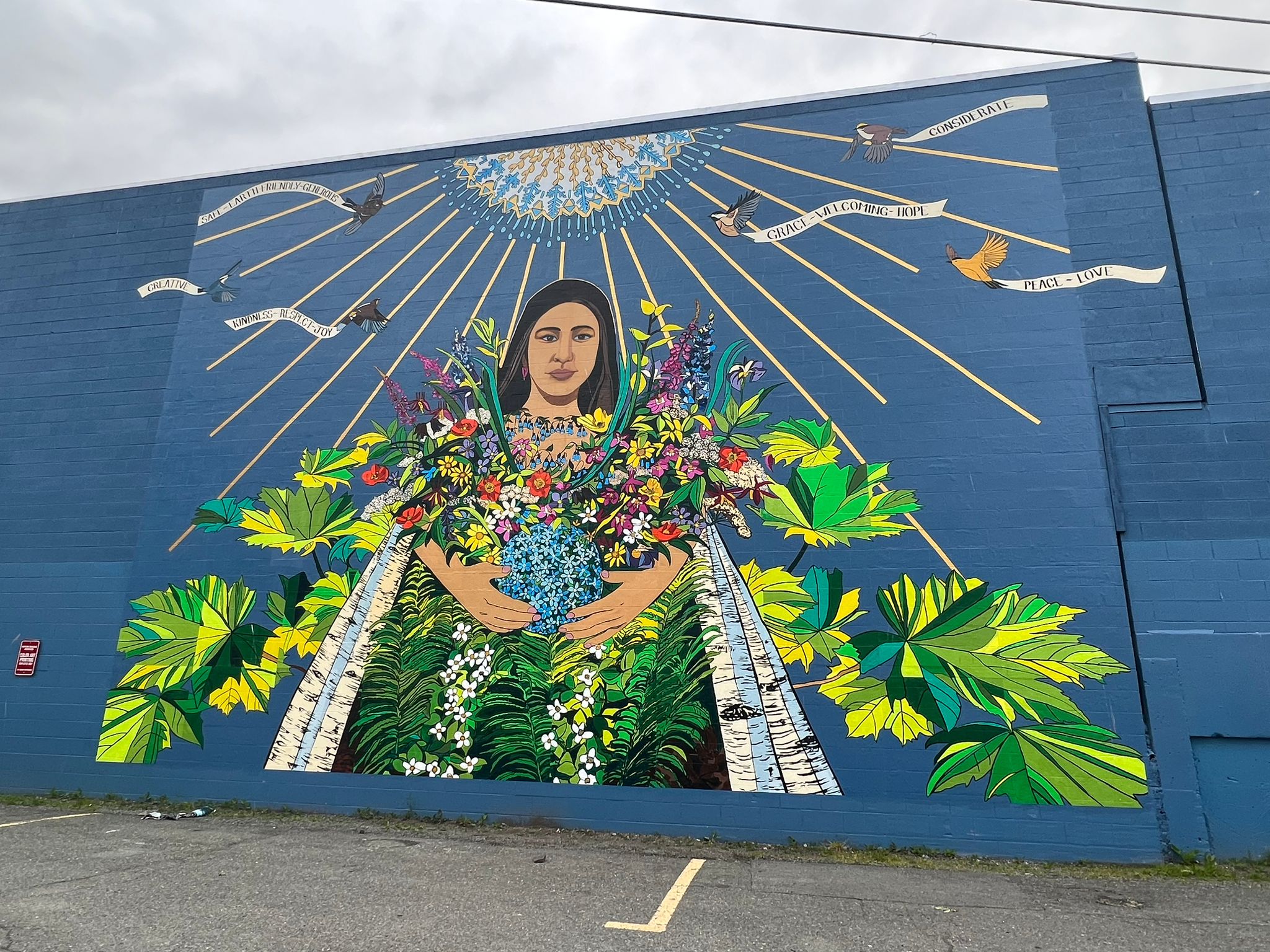The image shows a vibrant, outdoor mural painted on a dark blue wall, set against the backdrop of a cloudy sky and power lines overhead. The mural, located on the side of a building in Anchorage, Alaska, features a central figure of an indigenous Hispanic woman with long, dark hair pulled back. She is dressed in a robe made of green leaves and flowers, and holds a vase filled with various colored wildflowers across her bodice. Radiating behind the woman is a decorative sun made up of blue and yellow hues, which casts out rays adorned with ribbons. These ribbons bear inspirational words like "grace," "welcoming," "hope," "peace," "love," and "considerate." Birds can be seen flying among the sun’s rays, adding to the mural's dynamic and uplifting atmosphere. The mural is situated above a gray paved area, suggesting a parking lot or street below, emphasizing its urban environment. The overall style of the mural is photographic realism, capturing intricate details and textures.